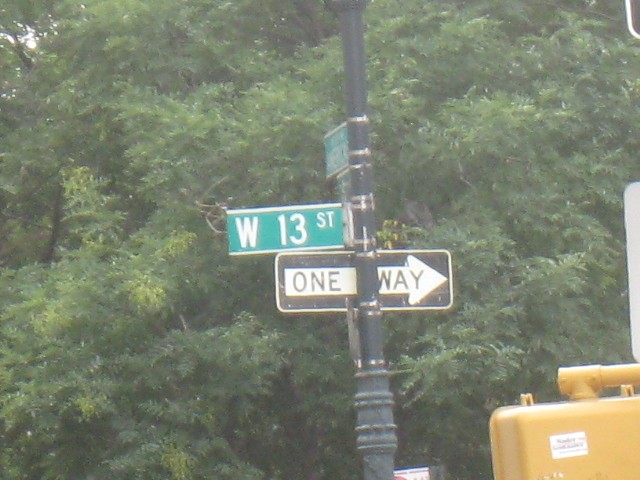A vibrant, color photograph features a central black metal pole adorned with multiple street signs. Dominating the pole is a green sign reading "West 13th Street." Directly below it, a black and white "One Way" sign points to the right. A third, barely visible sign, positioned perpendicularly to the other two, is angled in such a way that its text remains obscured. Surrounding the pole, lush trees form a verdant backdrop. The image appears to be taken from an elevated vantage point and is tightly cropped, excluding any visible sidewalk or street. The composition emphasizes the interplay of the signs against the natural greenery, capturing a slice of urban navigation amidst a leafy environment.